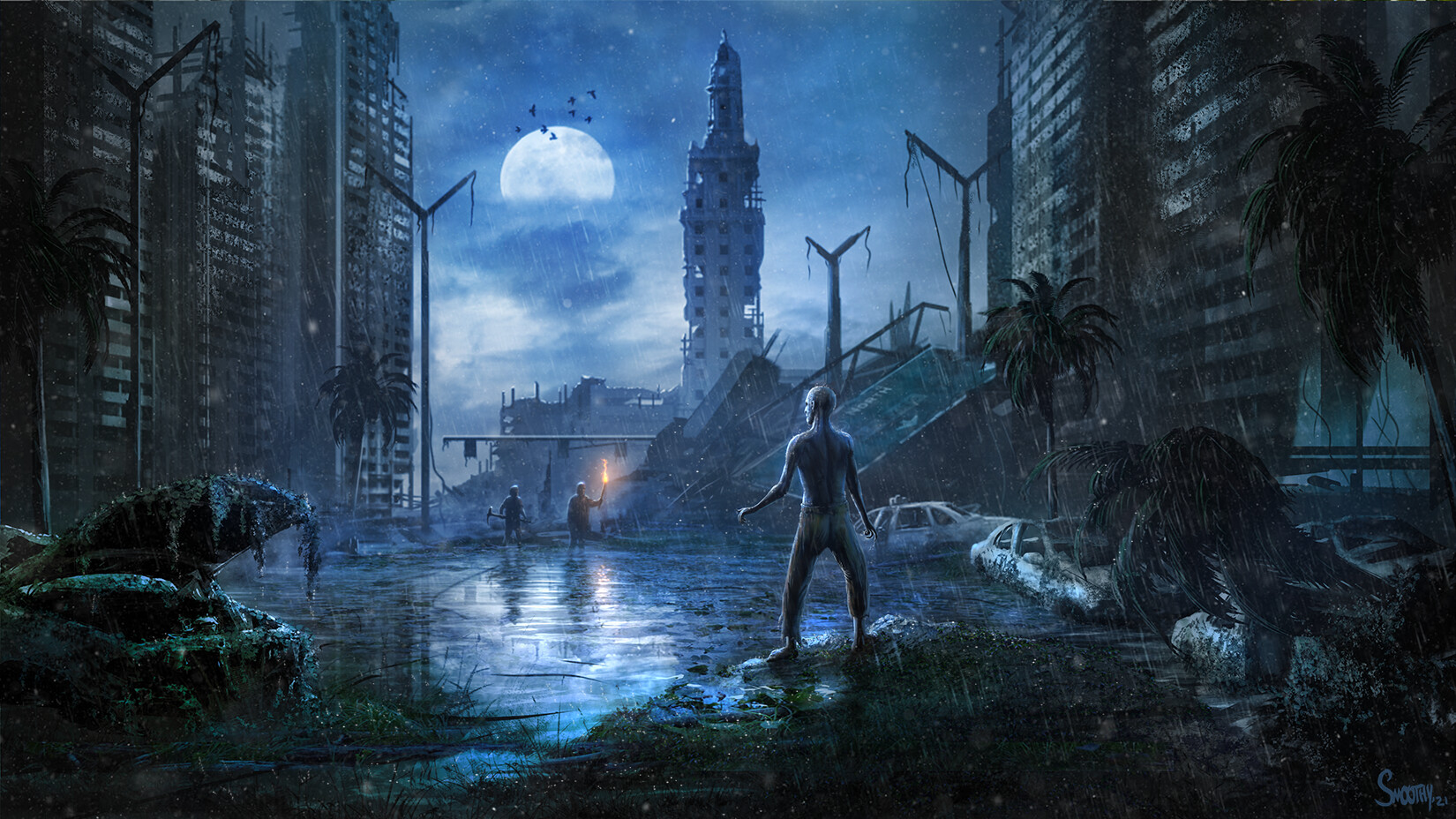This is a meticulously crafted graphic depiction of an apocalyptic urban setting, enveloped in a somber palette of blacks and blues, reminiscent of a video game scene. The backdrop reveals a partially clouded night sky illuminated by a half-moon, with dark birds circling ominously above. Among the ruins stand dilapidated buildings devoid of walls, their skeletal remains rising eerily against the sky.

In the foreground, a nude man stands atop rubble in an abandoned alleyway, appearing surprised and apprehensive. His gaze is fixed on two sinister figures approaching from the distance. One of these adversaries clutches a lit torch, casting an ominous glow, while the other wields an axe-like weapon, heightening the sense of imminent threat.

To the left of the scene, a frightening, large Komodo lizard-like creature roams, adding a further layer of menace. The cityscape around them shows signs of long-term decay, with grass and trees reclaiming spaces amidst the rubble and reflecting pools of water that mirror the moonlight. Abandoned vehicles and scattered debris further accentuate the desolation, occasionally interrupted by the eerie presence of figures in tattered hazmat suits, suggesting a desperate search for survival in this bleak, post-apocalyptic world.